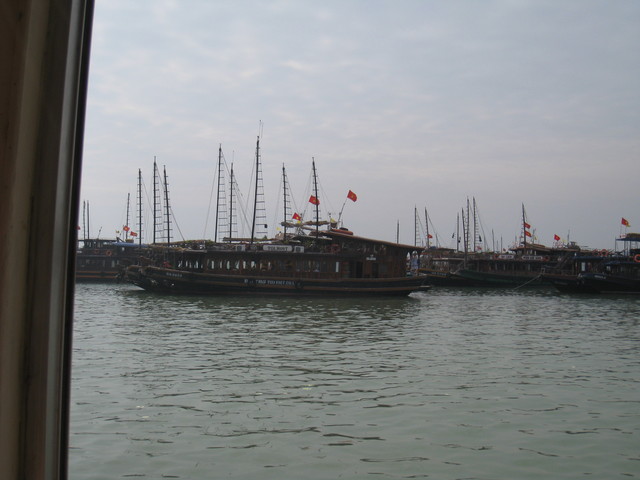In this landscape-oriented, rectangular image, captured from the window of another boat, we see a dreary yet serene maritime scene. Along the left border of the photo, a portion of a window frame is visible in brown and black hues, suggesting the image was taken from within a cabin. The bottom half of the image is dominated by still, clear, slightly greenish water that reflects the overcast sky. The top half showcases a predominantly light blue sky with patches of white clouds, creating a gloomy atmosphere.

Placing our focus on the horizon, a line of old-style boats fills the middle portion of the image. These wooden, one-story boats are dark brown and feature multiple windows along their sides. Each boat is equipped with masts, absent of sails, adorned only with ropes or strings hanging down for support. Protruding from the ends of the boats are long poles, each flying a vivid red flag, adding a splash of color against the muted palette of the scene. In the backdrop, we notice a collection of docks and additional maritime infrastructure, contributing to the overall feeling of a quiet, old marina on an overcast day.